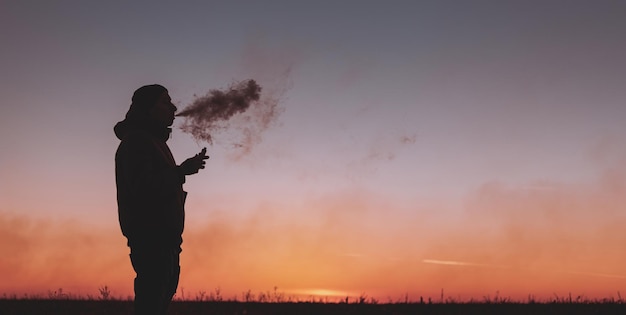In this photorealistic silhouette, a man stands in a grassy field at dusk, enjoying a smoke against the backdrop of a breathtaking sunset. He's holding something in his hand, possibly a cigar, pipe, or vape, as he exhales a large white cloud of smoke. The sky is a gradient of rich orange hues fading into the twilight's blue and purple tones, with the last vestiges of daylight illuminating the scene. His silhouette is featureless, save for the hint of long hair and the casual attire that suggests he might be wearing a hoodie with the hood down. The vibrant colors of the sunset and the detailed dark outlines of the grassy field, complete with scattered twigs and distant trees, create a tranquil yet evocative atmosphere.